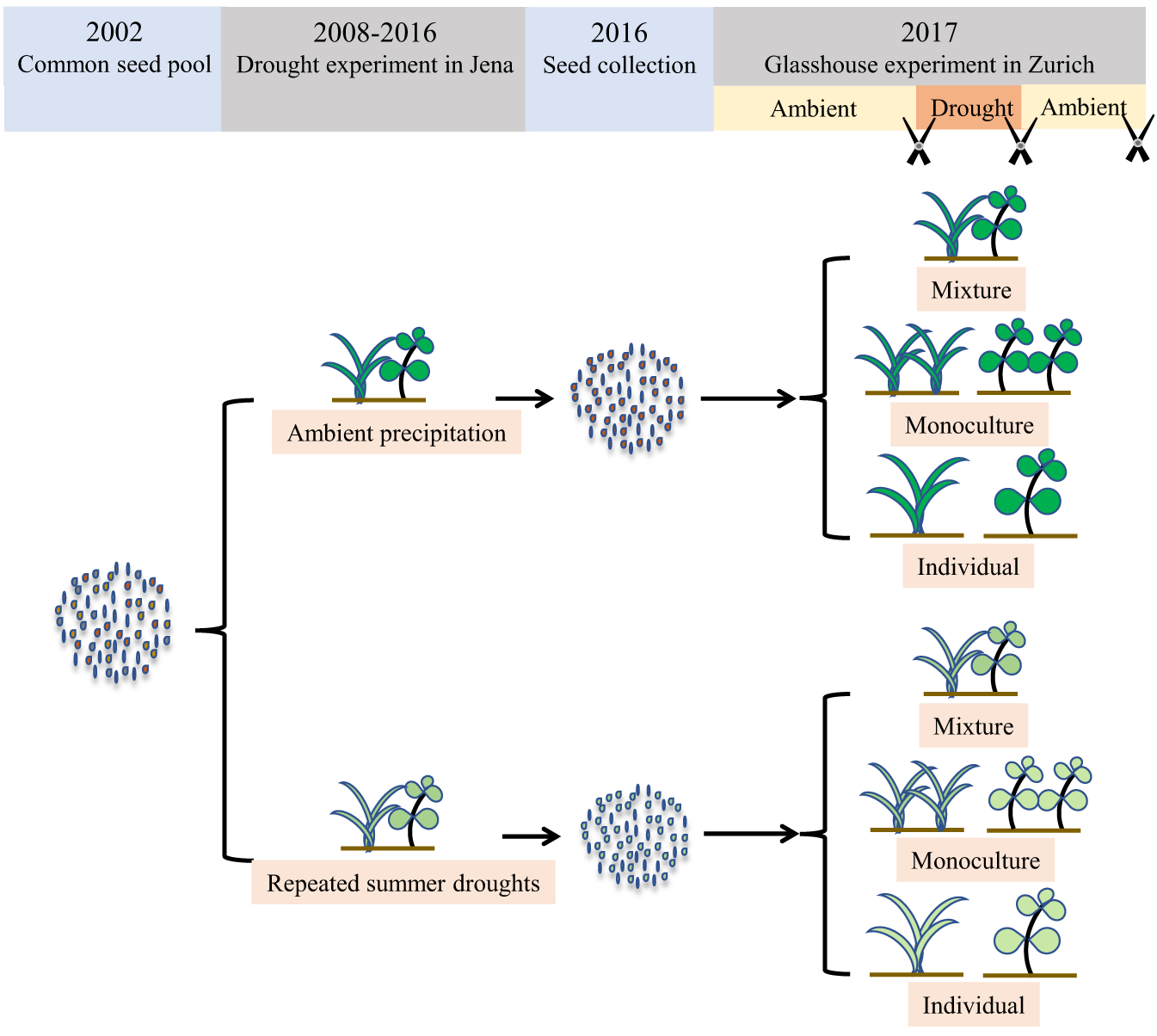This infographic provides a comprehensive timeline and experimental flowchart detailing the progression and effects of various seed propagation trials from 2002 to 2017. At the top, a timeline with alternating light blue and gray columns lists the key milestones: the "2002 Common Seed Pool," the "2008-2016 Drought Experiment in Jena," the "2016 Seed Collection," and the "2017 Glasshouse Experiment in Zurich." Directly below, the timeline is segmented into three labeled sections in yellow and orange, indicating different experimental conditions: "Ambient," "Drought," and "Ambient." 

The flowchart illustrates the developmental trajectory of seed lineages, starting from seeds on the left and progressing through different conditions and outcomes. Seeds under the "Ambient Precipitation" condition lead to three sowing strategies: "Mixture," "Monoculture," and "Individual." Similarly, seeds under "Repeated Summer Droughts" proceed through the same sowing strategies but result in visibly different plant growths. The seeds themselves are depicted with pink fillings turning hollow or white with blue borders under different conditions, highlighting the physical changes due to varying environmental stresses. The vibrant, healthy illustrations of plants at the top versus the grayish-green ones at the bottom further emphasize the contrasting outcomes of ambient conditions versus repeated droughts.